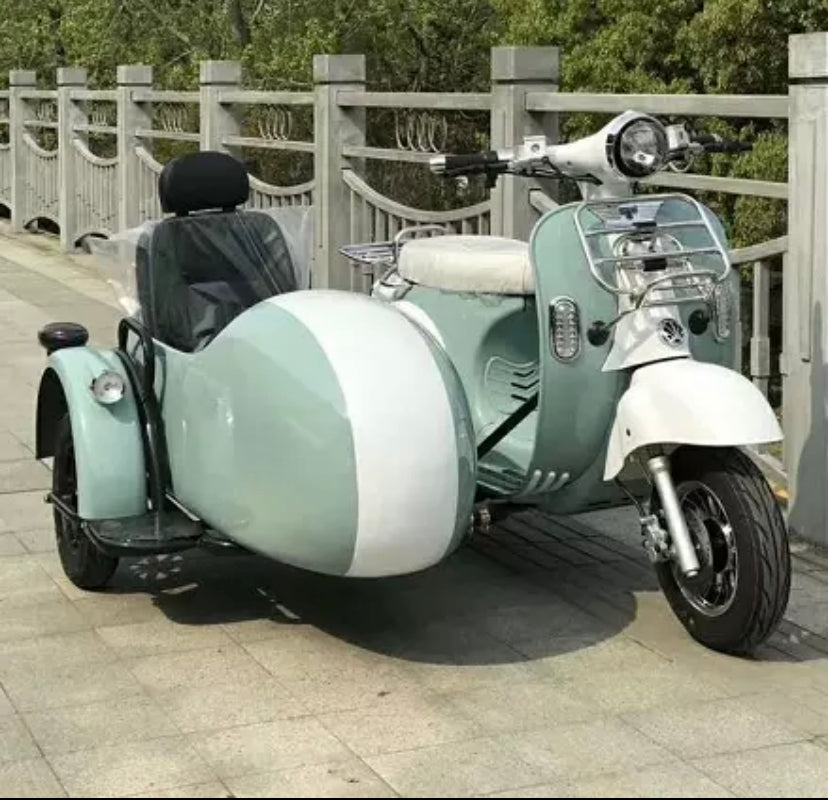In this image, we see a vintage-style motorcycle reminiscent of a Vespa, featuring a mint green color with white trim and black wheels. This motorcycle is equipped with a matching mint green sidecar that has a distinctive white line in the middle and a black seat, protected by a cover. The motorcycle, oriented towards the right, is parked on a bridge made of concrete pavers. The bridge has unique railings characterized by long, square-shaped posts connected by horizontal and curved ties with vertical slats in between. In the background, lush green trees suggest an outdoor daytime setting. No text or humans are present in the photo, emphasizing the classic design and serene surroundings.